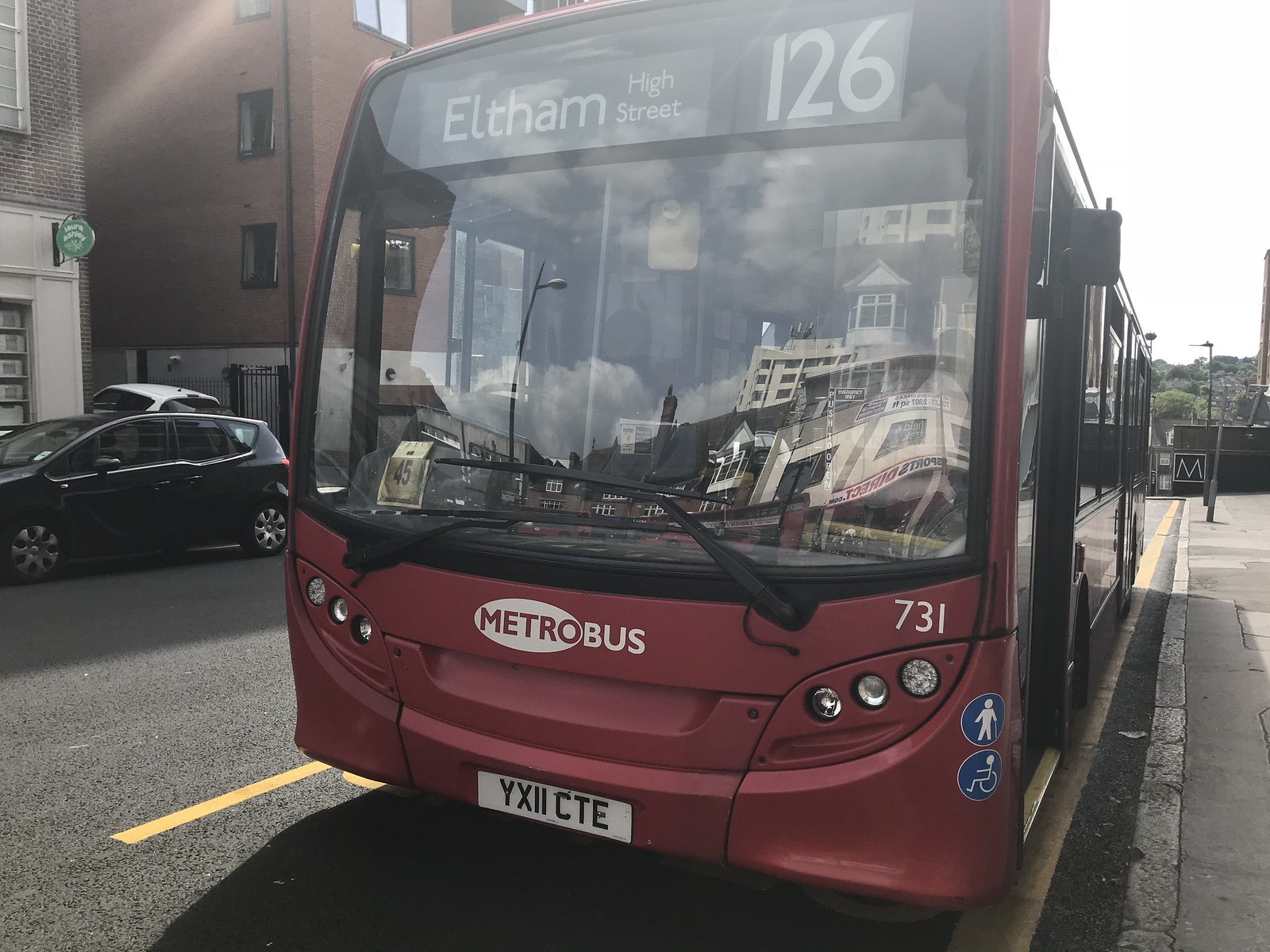An amber-colored bus bearing the route number 126 to Eltham High Street is parked along a city street under a sunny sky, casting a shadow onto the sidewalk. The bus features a large windshield with folded-down wipers, reflecting nearby buildings and shops. Prominently displayed at the top of the windshield is a black sign with white text indicating "Eltham High Street," adjacent to the route number "126." Below this, the Metro bus logo is visible, with "Metro" in red against a white oval and "bus" in white lettering. The front has three diagonal lights on each side, and a white license plate reading "YXIICTE" is mounted centrally on the bumper. Accessibility symbols for a person with a cane and a person in a wheelchair are present on the right side of the windshield, which also displays the number "731." The bus stands on a yellow line, its side adorned with windows extending approximately three-quarters of its length. Surrounding the bus are various city elements: to the left, a black car and a partially visible white car parked near a brick building, with another white-fronted brick building visible nearby. There’s also a green circular sign above the black car. In the background on the right, a black and white ground-level square displays a white "M," indicating a metro station or similar landmark, and some trees and fences are visible, suggesting a busy urban environment.